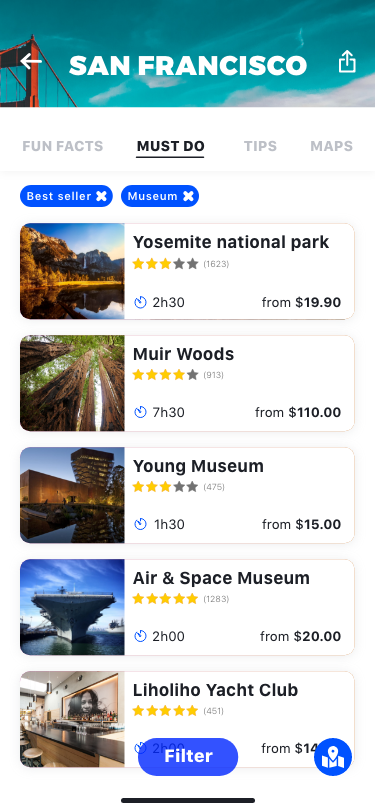The image captures a vibrant travel guide page for San Francisco. At the top, "San Francisco" is prominently displayed in crisp white text, flanked by a backward-facing white arrow and an upward-facing icon within a white square, all set against a blue background featuring a striking image of the iconic red Golden Gate Bridge. 

Below the header, a menu with a variety of tabs is visible: "Fun Facts" in gray, "Must Do" highlighted in black, "Tips" in gray, and "Maps" also in gray. The interface includes several tags such as "Bestseller" and "Museum."

Highlighted attractions are featured below:

- **Yosemite National Park:** Rated three stars, with an estimated visit duration of 2 hours and 30 minutes, and prices starting at $19.90.
- **Muir Woods:** A 7-hour and 30-minute excursion, costing from $110, showcasing an image of towering brown trees.
- **The Young Museum:** Also rated three stars, located 1 hour and 30 minutes away, with tickets starting at $15.
- **Air and Space Museum:** Rated five stars, situated 2 hours away with an entry fee starting at $20.
- **Holyo Yacht Club:** Also carrying a five-star rating, roughly 2 hours away. The accompanying image depicts a bar setting within a yacht club, accented by an artistic painting in the background. 

Each listing provides valuable insight into the variety of experiences available, with detailed time and cost estimates to help plan the perfect visit.